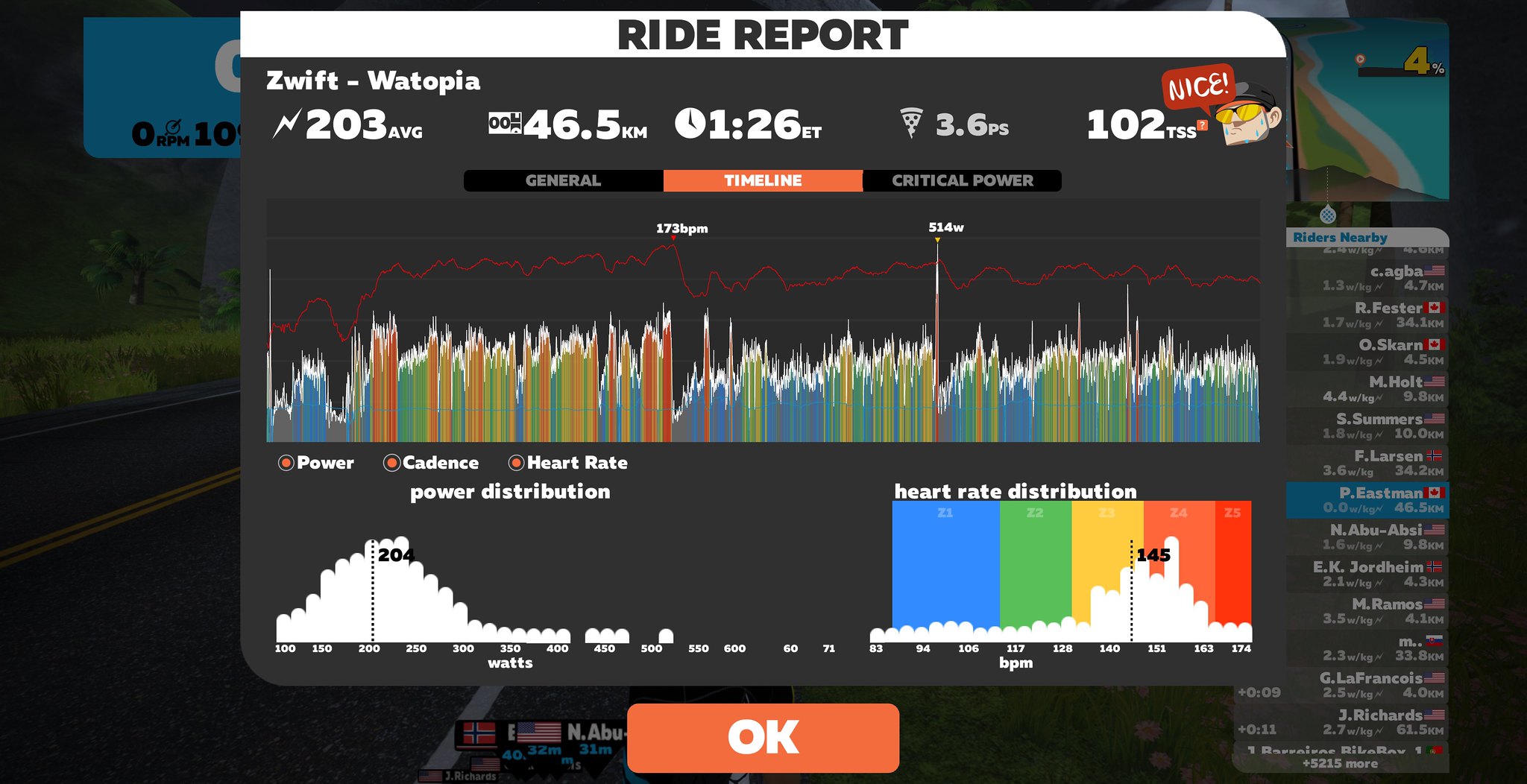The image displays a detailed screenshot of a graph within an app interface, labeled at the top in a white banner with black text, "RIDE REPORT, Zwift Watopia." Prominent metrics include 203 average, 46.5 km, 1 hour 26 ET, 3.6 PS, and 102 TTS. A cartoon character in the top right corner is accompanied by the word "Nice." Central to the image is a colorful bar chart, offering options such as general, timeline, and critical power. Below, additional buttons for power, cadence, and heart rate are present, alongside two more graphs: one for power distribution and the other for heart rate distribution. An orange rectangle labeled "OK" in white text sits at the bottom. The background hints at a road scene with grass on the sides, and to the right is a long list, possibly showing "RIDERS NEARBY" with corresponding country flags.